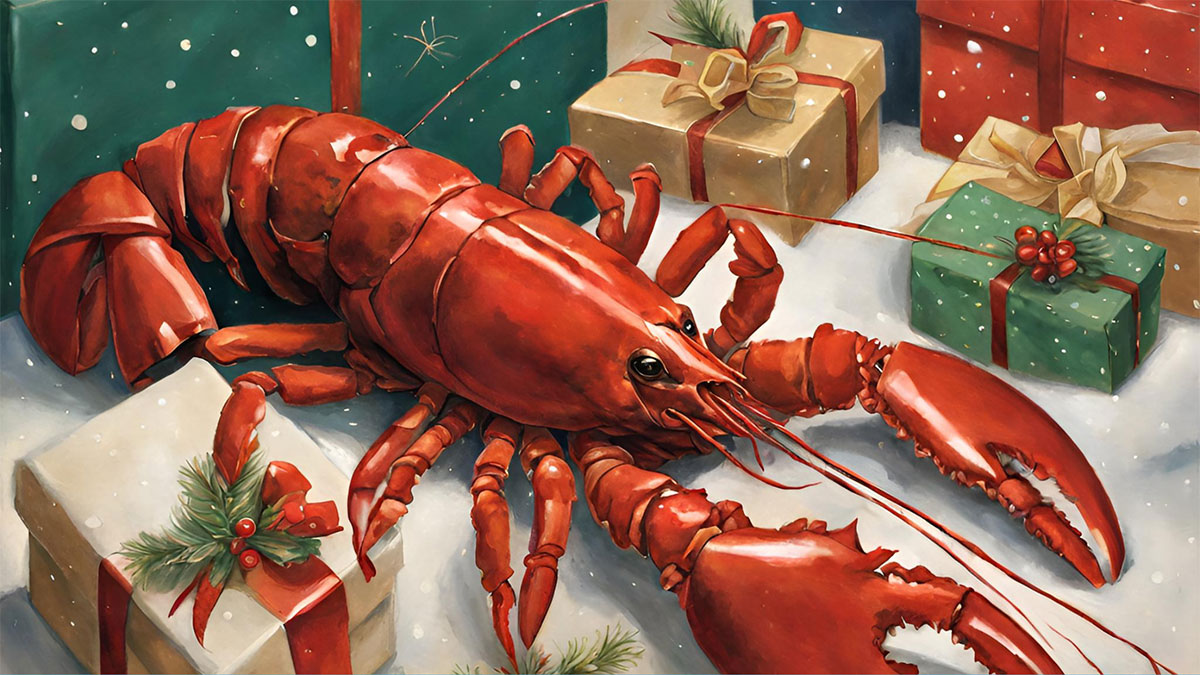This detailed drawing features an elaborate Christmas window display within a rectangular, horizontally-oriented frame. Central to the scene is a table sprinkled with fake, cottony snow, giving the setup an authentic winter feel. The backdrop shows a dark, teal-blue sky dotted with falling snowflakes, as visible through a display window. A spread of festively wrapped Christmas gifts—five in total—is meticulously arranged at the base. These presents, adorned with vibrant ribbons, greenery, berries, and red bows, come in a variety of colors: white, tan (two gifts), red, and green.

However, the most striking and unexpected element is a large red lobster placed among the presents. The detailed drawing captures the lobster in vivid detail, from its segmented body and tail to its prominent claws and antennae, topped off by its two black eyes. This unusual centerpiece creates an intriguing juxtaposition with the otherwise traditional holiday decorations, adding a touch of whimsy and surprise to the festive scene.